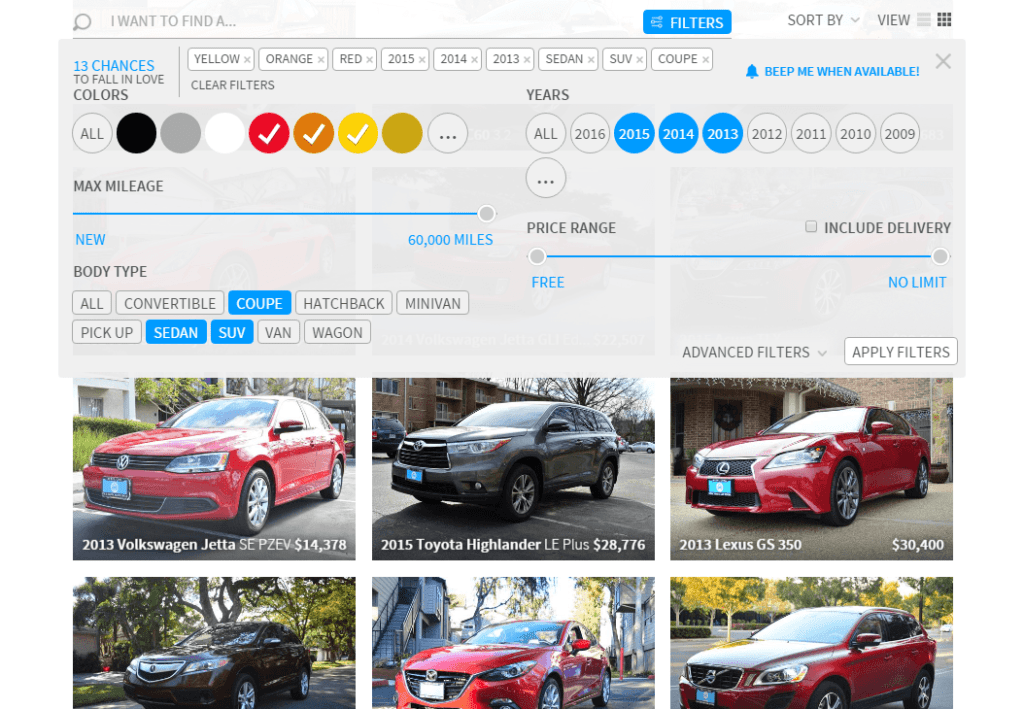A detailed screen capture from an online car marketplace shows an active search for vehicles filtered by multiple criteria. The selected filters include vehicle types such as coupes, sedans, and SUVs from the model years 2013 to 2016. Additionally, the search is refined to include cars with a maximum mileage of 60,000 miles, indicating that the desired cars are either new or lightly used. Most of the displayed cars are predominantly red, black, or silver, matching the specific color preferences set by the user. The brands visible in the search results include a mix of well-known manufacturers, such as Lexus and Volkswagen, among others. The displayed vehicles are described as generic-looking, blending seamlessly into typical urban roadscapes.